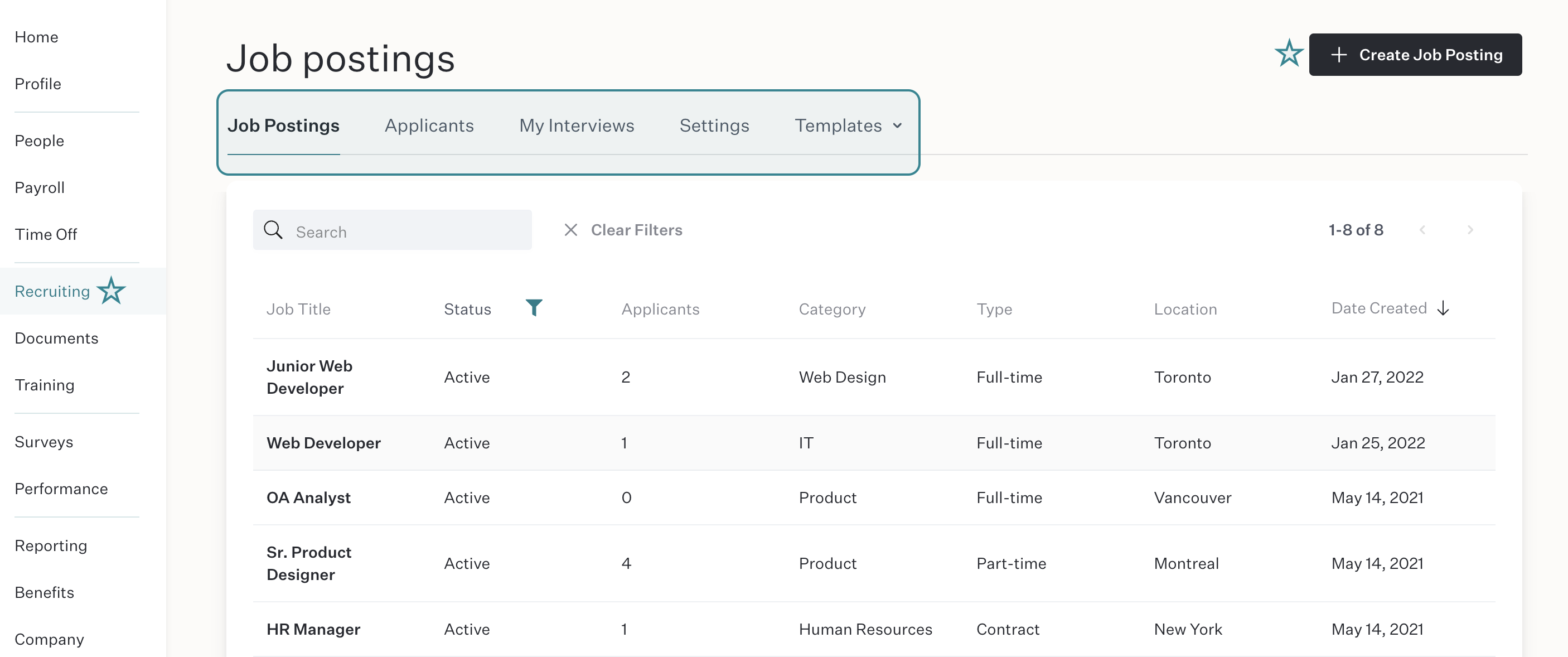**Detailed Website Screenshot Description:**

The image depicts a screenshot of a website with a vertical navigation pane on the left and a detailed main content area. The navigation pane contains the following options from top to bottom: Home, Profile, People, Payroll, Time Off, Recruiting (which is highlighted in green with a star beside it), Documents, Training, Surveys, Performance, Reporting, Benefits, and Company.

In the main content area of the page, the section titled "Job Postings" is prominently displayed. Within this section, a highlighted green-bordered area labeled "Hot" contains five items arranged vertically. The items are: 
- Job Postings (bold) 
- Applicants (gray font) 
- My Interviews (gray font) 
- Settings (gray font) 
- Templates (gray font).

Above these items, there is a search bar featuring a magnifying glass icon and the word "Search," followed by an "X" button labeled "Clear Filters."

Below the highlighted section, there is a comprehensive table encompassing seven columns with the following headers: Job Title, Status, Applicants, Category, Type, Location, and Date Created. Each column provides detailed information for various job positions:
1. **Junior Web Developer**:
   - Status: Active
   - Applicants: 2
   - Category: Web Design
   - Type: Full-time
   - Location: Toronto
   - Date Created: January 27, 2022

2. **Web Developer**:
   - Status: Active
   - Applicants: 1
   - Category: IT
   - Type: Full-time
   - Location: Toronto
   - Date Created: January 25, 2022

3. **OA Analyst** (repeated twice):
   - Status: Active
   - Applicants: 0
   - Category: Product
   - Type: Full-time
   - Location: Vancouver
   - Date Created: May 14, 2021

4. **Senior Product Designer**:
   - Status: Active
   - Applicants: 4
   - Category: Product
   - Type: Part-time
   - Location: Montreal
   - Date Created: May 14, 2021

5. **HR Manager**:
   - Status: Active
   - Applicants: 1
   - Category: Human Resources
   - Type: Contract
   - Location: New York
   - Date Created: May 14, 2021

At the very top above the "Date Created" column, a label indicates that the page displays records "1 through 8 of 8." Additionally, a small funnel icon is present next to the "Status" column header, suggesting filter options are available for this column.